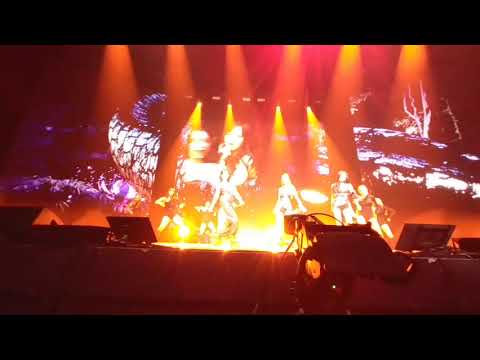The photograph captures a concert scene with an overall reddish hue dominating the image. The stage, awash in red light, is highlighted by at least six distinct shafts of light descending from above, with smaller orange shafts rising from below, targeting the performers on stage. The performers appear to be well-toned women, dressed in elaborate but somewhat scantily-clad costumes, engaged in dance rather than playing instruments, their features obscured by the vivid lighting.

In the background, there's a large screen displaying what appears to be a mix of artistic visuals, possibly including a somewhat realistic yet abstract representation of trees and serpentine scales. The upper and lower edges of the photo are framed with black bands, adding to the dark, intense atmosphere of the scene.

The foreground contains various technical equipment such as computers, speakers, and possibly drum monitors, hinting at the complexity of the stage setup. The left and right edges of the photo show a gradient of colors, from black in the lower sections to a blend of red, purple, and blue hues higher up, adding to the immersive and vibrant visual experience of the concert.